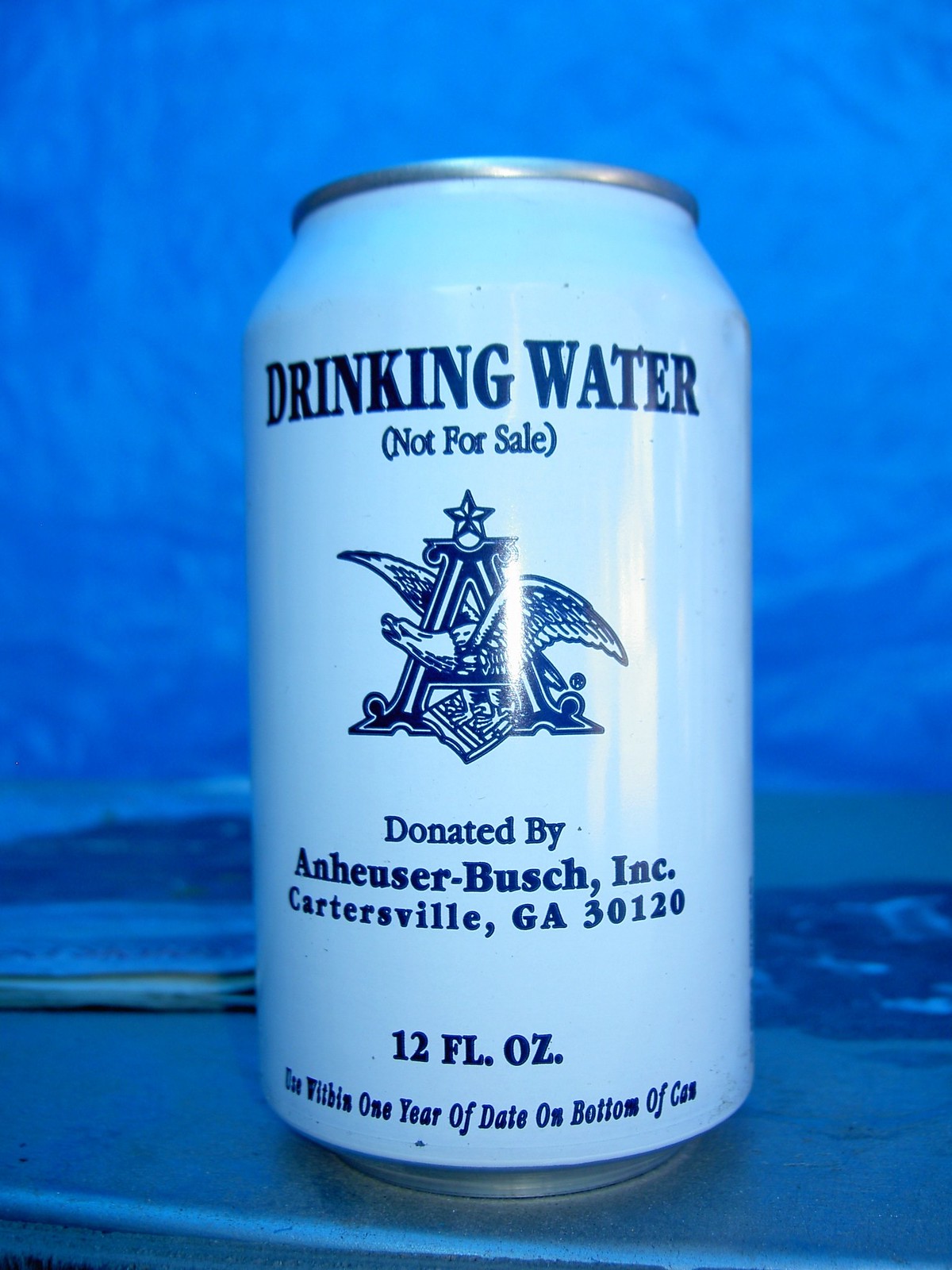This detailed photograph captures a 12 fluid ounce white aluminum can of drinking water, prominently featuring blue lettering. The can's top and bottom are rimmed with silver aluminum. Centered within the photo and resting on a blue surface, the can stands out against a bright, slightly out-of-focus blue background that resembles crinkled cloth or paper. The can is emblazoned with "Drinking Water" in large navy blue print, followed by "Not for Sale" in parentheses below. The distinctive Anheuser-Busch logo, an 'A' with an eagle's wings extending from it, is visible beneath the text. Further down, the can states "Donated by Anheuser-Busch, Inc., Cartersville, Georgia, 30120." Towards the base of the can, "12 Fluid Ounces" is printed, and near the bottom is a partially obscured message indicating the water should be consumed within one year of the date stamped on the can’s bottom. No people or additional identifying features accompany the can in the photograph.